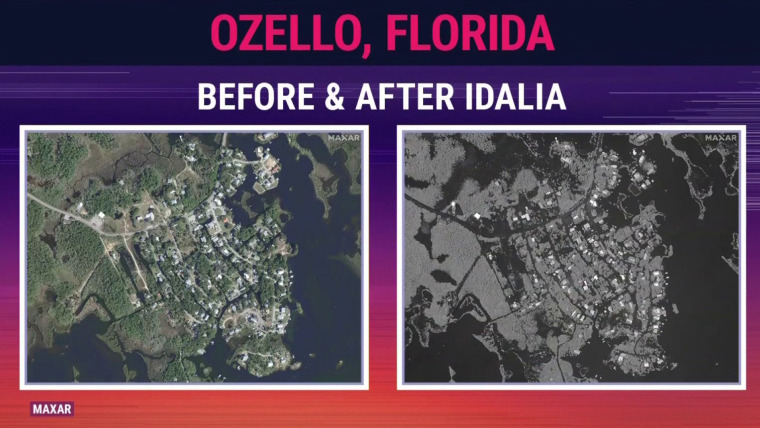The image is a detailed screenshot from a computer, showcasing Ozello, Florida, before and after the hurricane Idalia. At the top of the image, the text "OZELLO, Florida" appears in pink against a black background, followed by another line in white text against a purple background that reads "before and after Idalia." Below this heading, two side-by-side aerial photographs with white borders are set against a coral-colored background. The left photograph displays the town before the hurricane, featuring lush greenery, various buildings, multiple water bodies including a large bay, a river, and small ponds, as well as visible roads and development. In stark contrast, the right photograph reveals the aftermath: the vibrant greenery has been replaced by a desolate gray landscape, with no visible trees, many buildings destroyed, and extensive flooding, which has transformed smaller ponds into expansive lakes. The devastation is clear, with the town appearing largely obliterated and muddy. In the lower left-hand corner of the image, the letters "MAXAR" suggest the involvement of a satellite imaging company.